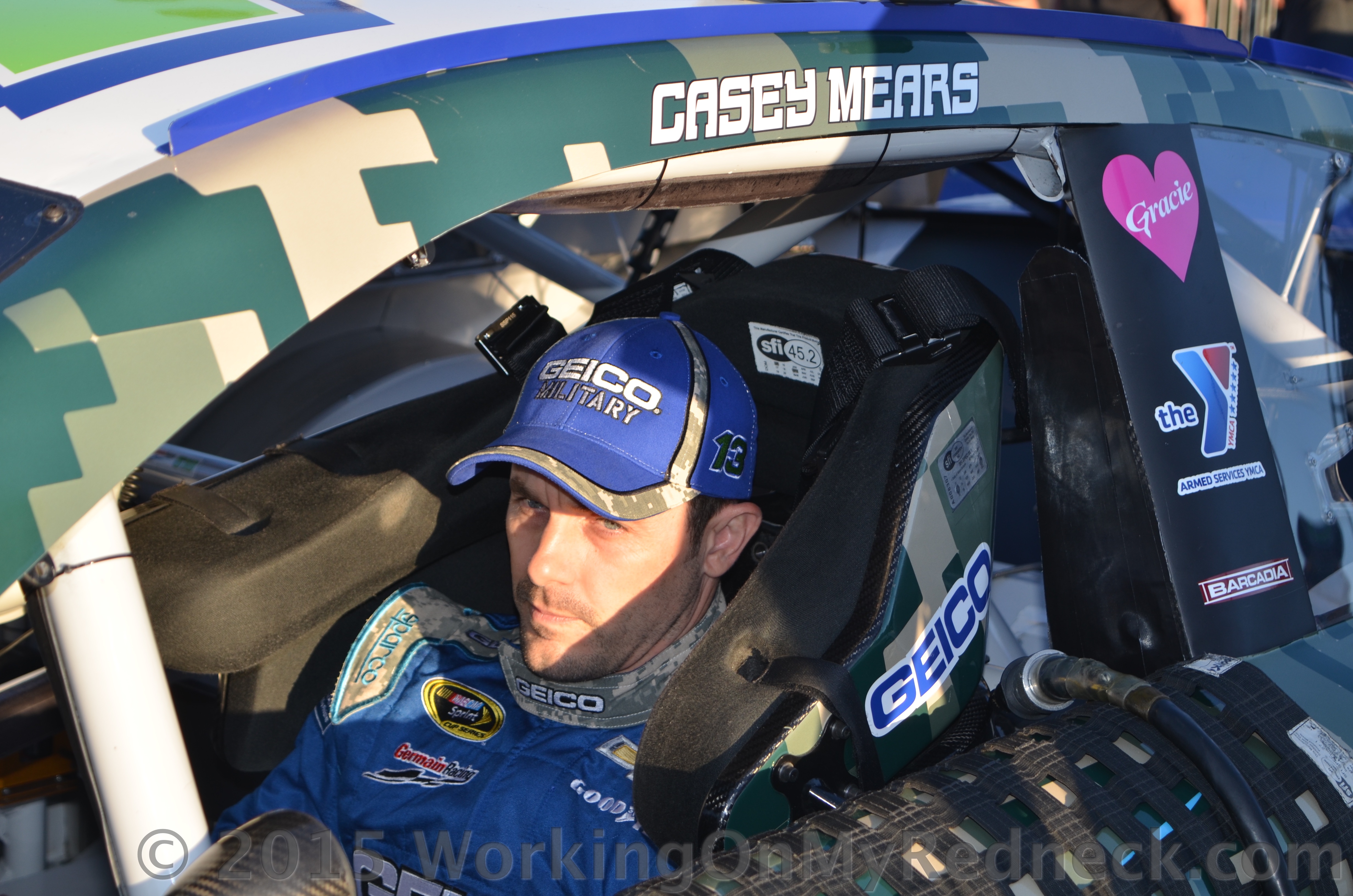In this detailed photograph, NASCAR driver Casey Mears is centrally positioned inside his race car. The car, displaying a combination of light teal green, white, and blue, prominently features Casey Mears' name in green camouflage print on the top panel above the driver’s side. Mears is seated in the driver's seat, enveloped by a padded seat that bears the Geico logo. He is dressed in a blue racing suit adorned with multiple sponsor logos, including Goodyear and Geico. Completing his racing attire, Mears dons a blue and white Geico Military hat, which also features the number 13. On the A-pillar of the car, next to the window, there is a red, white, and blue YMCA sticker, as well as a pink heart decal with the name "Gracie" inscribed in the center. Mears' expression appears neutral or perhaps slightly discontented as he looks out from his car. A copyright symbol at the bottom of the image notes "2015 working on my redneck.com."